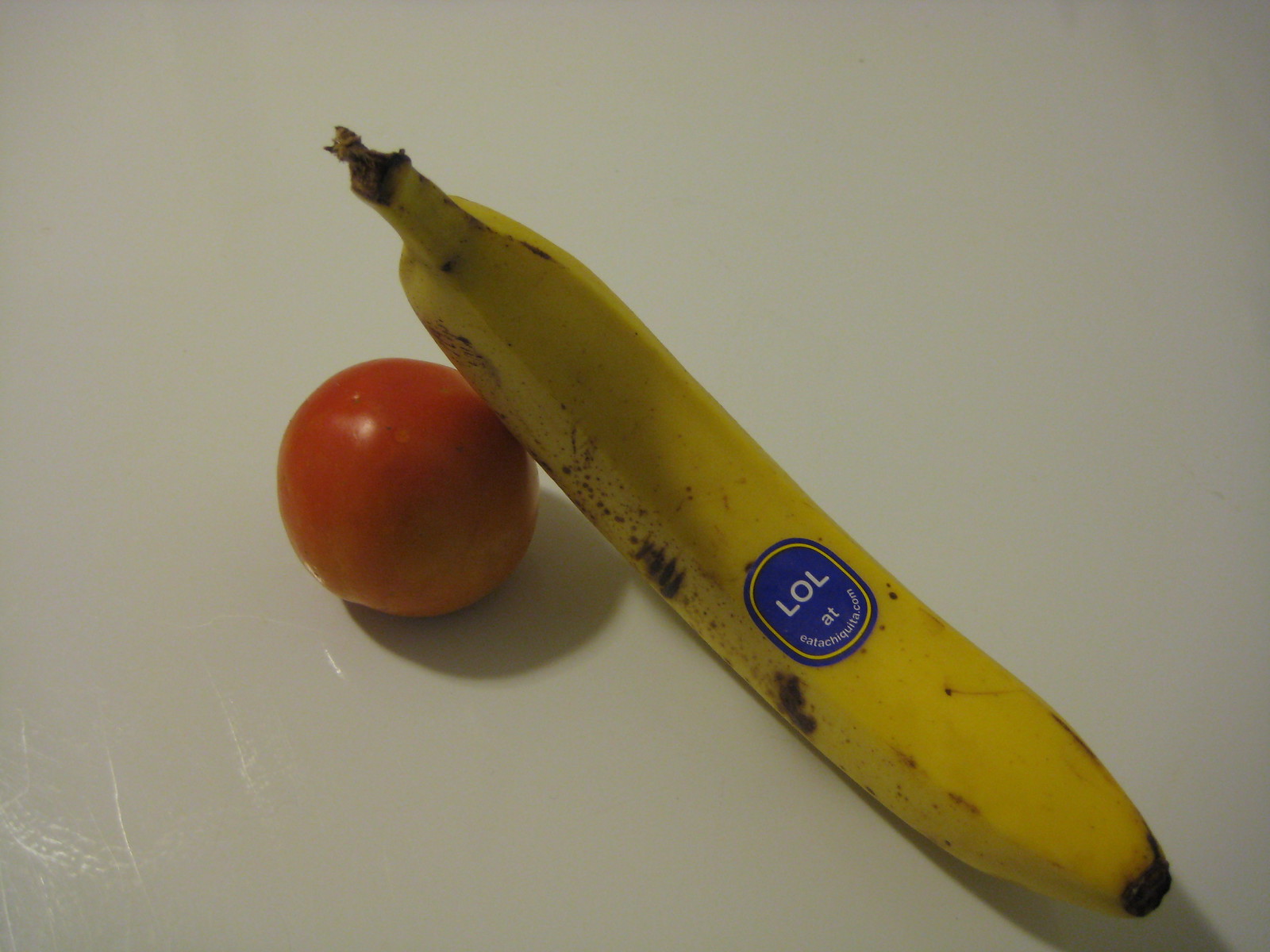In the image, a ripe banana is seen leaning against a fresh tomato on a plain white surface, possibly a table or countertop with no visible textures or indentations. The banana, which appears perfectly ripe and ready to eat, features a small sticker that reads "lol" and "eatachiquita.com." The bright red tomato, untouched and ripe, serves as a makeshift support for the banana, preventing it from toppling over. The scene is minimally detailed, with only the shadows giving any hint of depth or dimension to the otherwise simple setup.